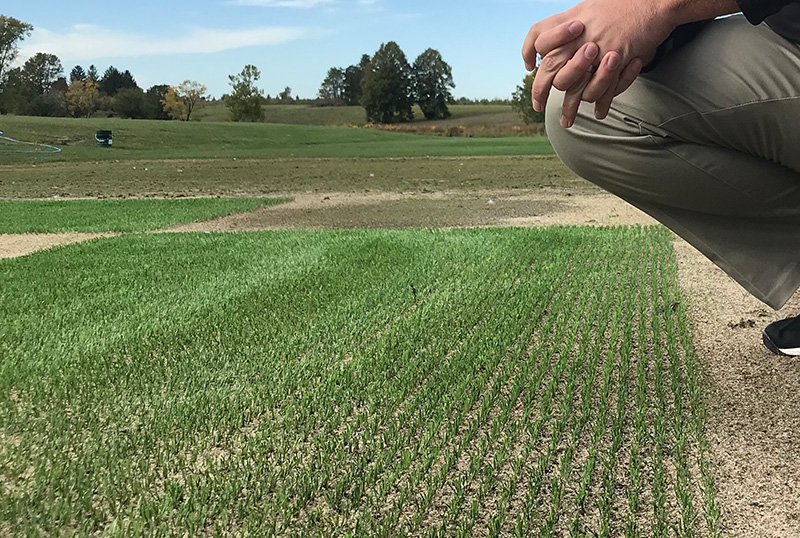The photograph captures a detailed outdoor scene of a farming landscape under a clouded sky. At the center, we see a nursery bed with rows of tiny, vibrant green plants beginning to sprout from the ground, organized meticulously into squares. These squares appear to be part of a crop rotation system, with some squares left barren to rest and rejuvenate the soil. In the foreground, notably on the right-hand side, a man is squatting down close to the sprouting plants. His attire includes tan khaki pants and black shoes, and although only his knee, thigh, calf, and clasped hands resting on his knee are visible, he appears to be inspecting the young plants with keen interest. The scene extends to a plain background with scattered trees and bushes, mostly in shades of green, adding to the serene agricultural setting.